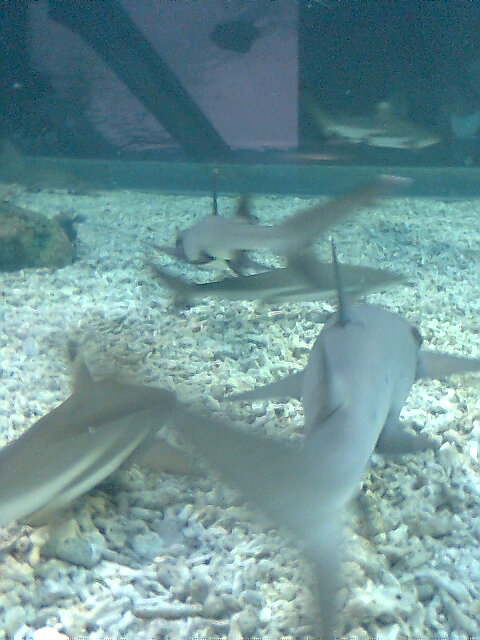This image captures an underwater scene from inside a rather blurry shark aquarium tank. The focus is on six juvenile sharks of varying sizes, identifiable by their gray backs and white undersides, swimming at different speeds. Most of these sharks are oriented away from the camera, displaying their distinctive dorsal fins while masking their heads. The tank's floor is covered with a mix of small smooth stones, chunks of white coral, some larger rocks, and patches of sand. An angled bar and a green line are noted at the bottom edge of the glass, alongside a bluish fish that hovers a foot or two above the tank floor. A pink object and a mirrored surface on the opposite side of the tank reflect the sharks' movements, adding depth to the image. In the background, there is a faint purple hue and a blurred spectator can be seen outside the tank, adding to the aquarium setting.